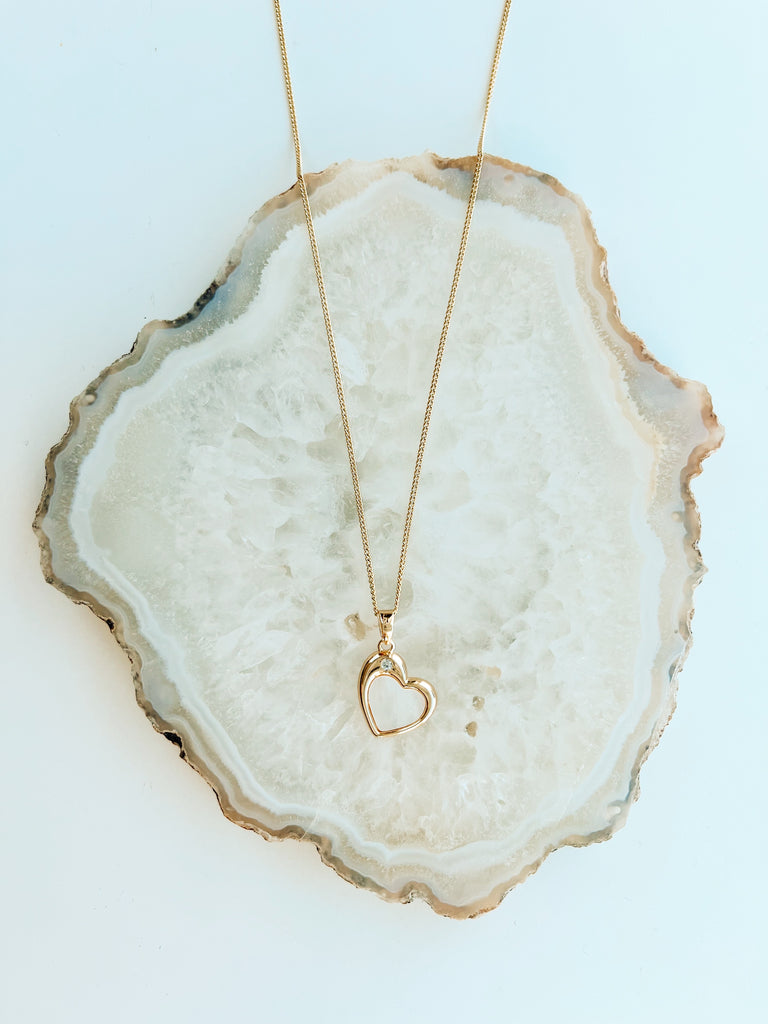The detailed photograph, framed in portrait orientation, showcases a beautifully polished cross-section of a geode, serving as an elegant display backdrop against a soothing pale aqua-blue background. The geode, primarily white with sections of off-white, gray, and dark brown bands, exhibits a mesmerising, natural concentric pattern akin to mother-of-pearl. Towards its edges, it darkens to a rich brown, creating a striking contrast to the lighter inner sections.

Resting atop this geode is an exquisite gold necklace. The delicate and long chain, composed of small, linked circles, highlights a hollow heart pendant. Positioned elegantly within the heart's hollow is a single, sparkling diamond, adding a touch of sophistication to the minimalist design. The simplistic beauty of the necklace against the natural allure of the geode suggests that this photorealistic image is likely aimed at showcasing the jewelry for potential buyers.